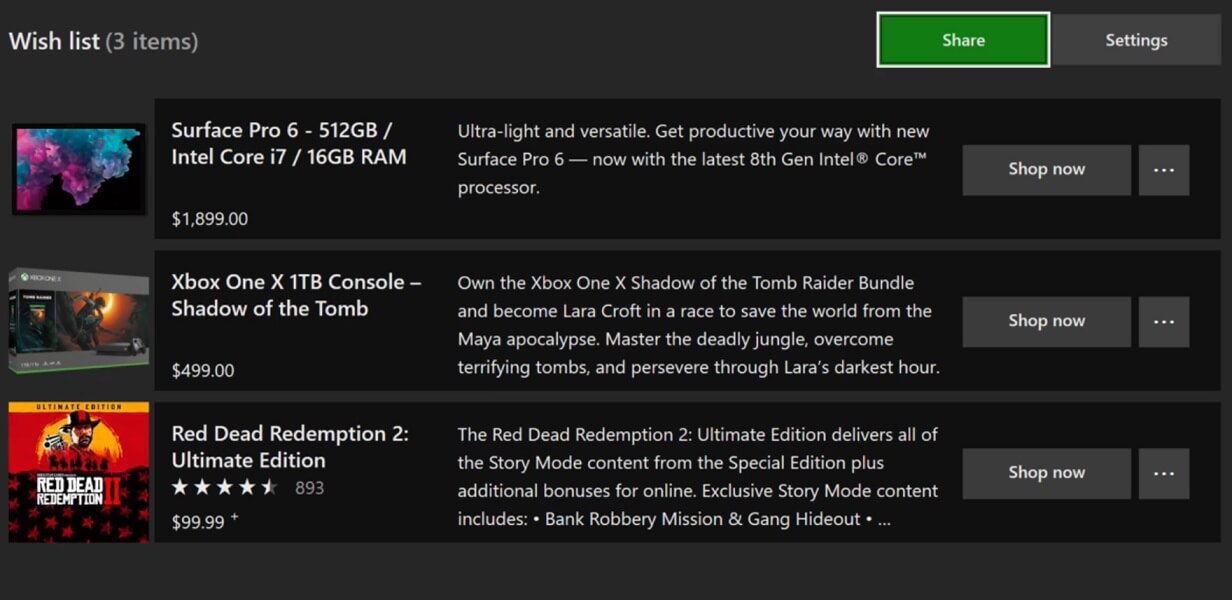The image showcases a section of an online shopping interface featuring a watchlist with three items and several action buttons. On the top right, there is a green "Share" button with white text, looking as if it's about to be clicked, followed by a "Settings" button in white text.

1. **Surface Pro 6**:
   - **Visual**: A product image resembling a purple and bluish cloud with a smoke effect.
   - **Title**: Surface Pro 6 - 512GB / Intel Core i7 / 16GB RAM
   - **Price**: $1,899.00
   - **Description**: "Ultra-light and versatile. Get the product your way with the new Surface Pro 6, now with the latest 8th Gen Intel Core processor."
   - **Actions**: "Shop Now" button followed by an ellipsis (three dots).

2. **Xbox One X Console - Shadow of the Tomb Raider Bundle**:
   - **Visual**: An image of a game box with a distinct Shadow of the Tomb Raider cover.
   - **Price**: $499.00
   - **Description**: "On the Xbox One X Shadow of the Tomb Raider bundle, become Lara Croft in a race to save the world from the Mayan apocalypse. Master the deadly jungle, overcome terrifying tombs, and persevere through Lara's darkest hour."
   - **Actions**: "Shop Now" button followed by an ellipsis (three dots).

3. **Red Dead Redemption 2: Ultimate Edition**:
   - **Visual**: A cover featuring a cowboy with a red hat against a yellow sun background. A yellow line at the top reads "Ultimate Edition" in black letters, and "Red Dead Redemption" in white letters with the number "2" in red.
   - **Rating**: 4.5 stars from 893 reviews.
   - **Price**: $99.99
   - **Description**: "Red Dead Redemption 2: Ultimate Edition delivers all of the story mode content from the Special Edition plus additional bonuses for online. Exclusive story mode content includes a bank robbery mission and gang hideout."
   - **Actions**: "Shop Now" button followed by an ellipsis (three dots).